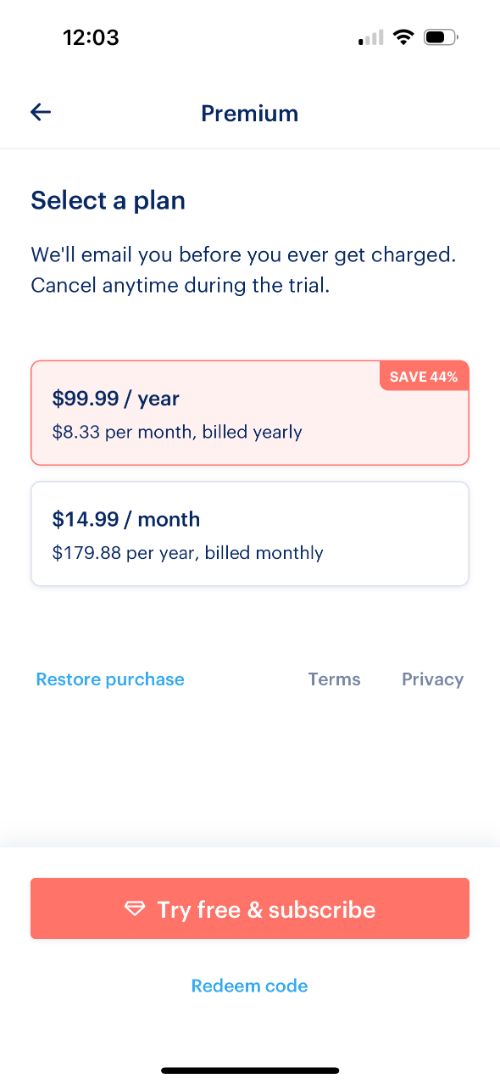The image captures a screenshot of a phone displaying a subscription plan selection page for a premium service. 

At the top, the heading reads "Premium" with the current time shown as 12:03. Below the "Premium" heading, a secondary heading says, "Select a plan." An informational note follows, stating, "We'll email you before you ever get charged. Cancel any time during the trial."

A pink rectangle prominently displays the first subscription option: "$99.99 a year," and clarifies the cost further with "$8.33 per month billed yearly." A pink flash in the corner highlights a "Save 44%" discount.

Below this, the monthly subscription option is presented: "$14.99 a month," totaling "$179.88 per year billed monthly."

At the bottom, a pink button invites users to "Try Free and Subscribe." Additionally, a link to "Redeem Code" is provided.

Above these options, several buttons offer more details and functionalities, labeled "Restore Purchase," "Terms," and "Privacy," for users seeking more information or needing to restore previous purchases.